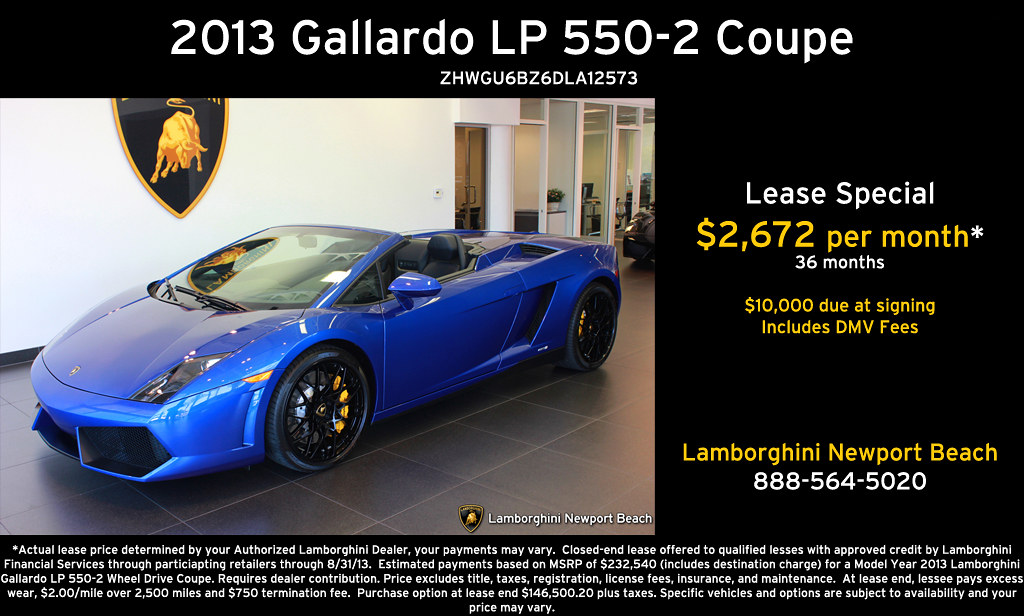This image is an advertisement for a 2013 Gallardo LP 550-2 Coupe on a black background. At the top, in white lettering, it reads "2013 Gallardo LP 550-2 Coupe." The lower left corner features a striking, bright blue Lamborghini sports car with black wheels, yellow brake calipers, and a shiny, convertible body. The vehicle is displayed on a tiled showroom floor with a white wall behind it, and the Lamborghini logo is visible on the left side in the background. The right side of the ad, against the black backdrop, highlights the lease special offer: "$2,672 per month for 36 months, $10,000 due at signing including DMV fees." The dealership details "Lamborghini Newport Beach" and the contact number "888-564-5020" are also provided. The fine print mentions the dealer's terms and conditions for varying payments.